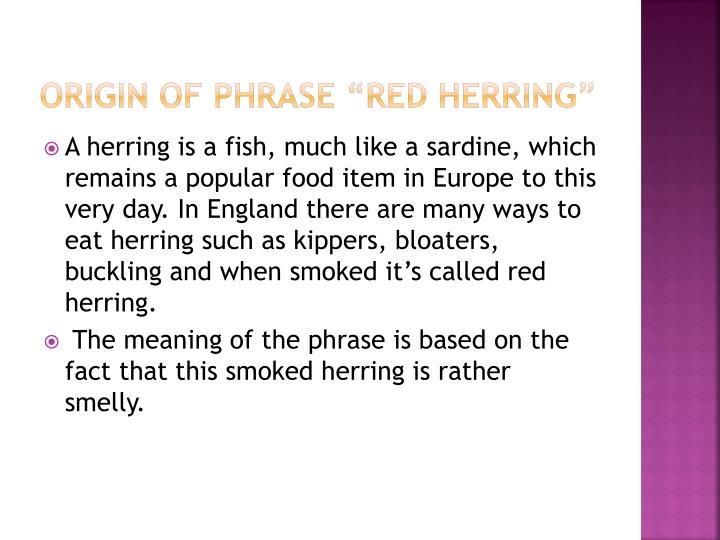The image resembles a PowerPoint slide with a predominantly white background. To the right side of the slide, there is a striking rectangular panel featuring a gradient that transitions from dark purple at the top to light purple at the bottom. The heading, "Origin of Phrase: 'red herring'," is prominently displayed at the top in transparent, graduated lettering that fades from white to dark yellow. Below the heading, there are two bullet points within purple circles, which are also outlined in purple. 

The first bullet point explains that a herring is a fish similar to a sardine, a popular food item in Europe. It details various traditional ways to eat herring in England, such as kippers, bloaters, and buckling, noting that when herring is smoked, it is referred to as red herring. The second bullet point clarifies that the phrase "red herring" is derived from the fact that smoked herring has a rather strong, smelly odor. All text within the bullets is black. 

Overall, the slide blends informative content about the origin and meaning of the phrase "red herring" with a visually engaging design, combining textual details and gradient color schemes.